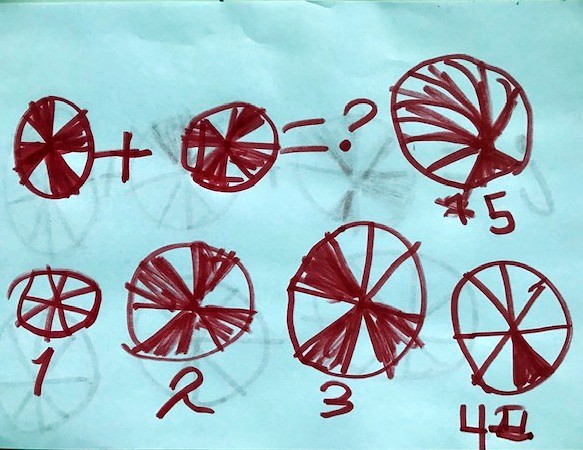This image features a piece of paper with a bluish tint, possibly caused by lighting or the paper's inherent color. The paper is covered in various sketches made with a reddish-brown marker. 

In the top row, there are several drawings and symbols:
1. A solid, thick-lined circle.
2. A plus sign followed by another similar solid circle.
3. An equals sign leading to a question mark.
4. A larger circle filled with crisscrossing lines.
5. Beneath this chaotic circle, a number seven is visible but has been crossed out and replaced with the number five.

The bottom row contains four more circles, each distinct in its pattern, yet all maintaining the theme of scribbled lines:
1. The first circle is labeled with the number one and features thick, filled-in lines.
2. The second circle, marked with a two, also contains thick scribbles.
3. The third circle, designated with the number three, continues the pattern.
4. The fourth circle, labeled with the number four, shows evidence of an initial mistake in the number's rendering, which has been corrected.

The varying thicknesses of the lines and the mix of filled-in and sparse scribbles demonstrate diversity in the patterns while maintaining overall unity in the theme.